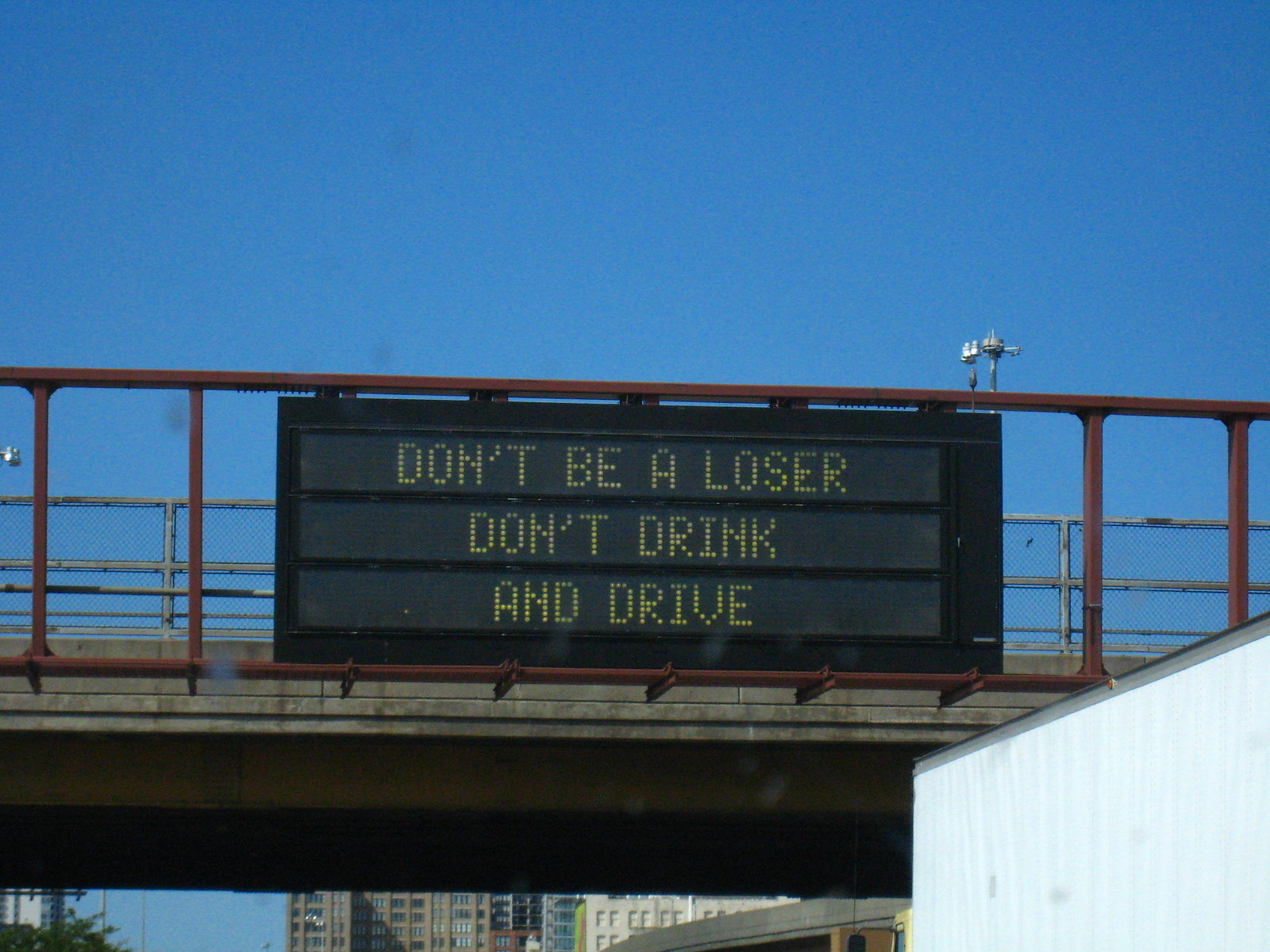In the image, a bright daylight scene captures a clear blue sky as the backdrop for a detailed view of a pedestrian bridge, prominently featuring brown rails on one side and gray rails on the opposite. The bridge is equipped with tall fences to prevent any interference from pedestrians. Dangling in the center of the bridge is a large black digital sign displaying a cautionary message with yellow dotted text. The sign's three lines read: "DON'T BE A LOSER," "DON'T DRINK," and "AND DRIVE." Below this bridge, we see the highway with the side of a white container truck and a yellow truck cabin visible in the lower right corner of the frame, accompanied by a hint of greenery in the lower left. Off in the distant background, partially obscured by the bridge's structure, there are urban buildings with many windows, suggesting modern apartment complexes. The photograph is well-lit and sharply focused, emphasizing the bright, clear day.